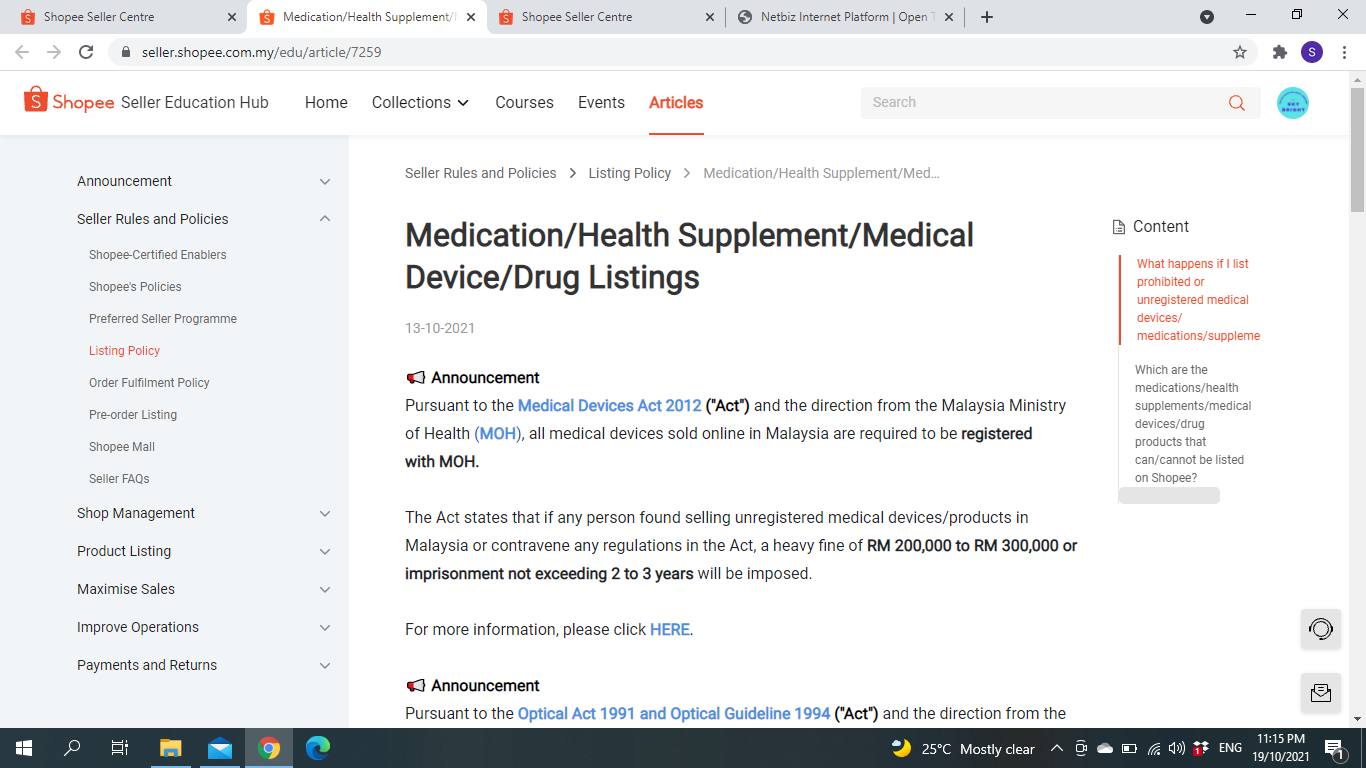The image depicts a screenshot of a web browser with four tabs open at the top. The active tab is titled "Medication and Health Supplement," and the full URL in the address bar is "seller.shopee.com.my.evu.article.7259." The website displayed belongs to Shopee and prominently features the Shopee logo—a shopping bag with an 'S' in orange.

The webpage header reads "SHOPEE Seller Education Hub" with a navigation menu including options like Home, Collections, Courses, Events, and Articles, accompanied by a search bar on the right-hand side.

On the left-hand side, set within a grey bordered panel, there are various categories listed, such as Announcements, Sellers, Rules, and Policies, under which several subcategories are expanded, including Shopee Certified Enablers, Shopee Policies, Preferred Seller Program, Listing Policy, Order Fulfillment Policy, Pre-Order Listing, Shopee Mall, Seller FAQs, Shop Management, Product Listing, Maximize Sales, Improve Operations, and Payments and Returns.

The primary content area on the right, set against a white background, is focused on "Seller Rules and Policies," specifically the "Listing Policy" for "Medication, Health Supplements, Medical Device, and Drug Listings." An announcement highlights pertinent regulations under the Medical Devices Act 2012 and directives from the Malaysian Ministry of Health, noting that all medical devices sold must be registered with the Ministry of Health. Failure to comply may result in severe penalties, including a fine ranging from RM 200,000 to RM 300,000 or imprisonment not exceeding two to three years. The page also provides a clickable link for more information.